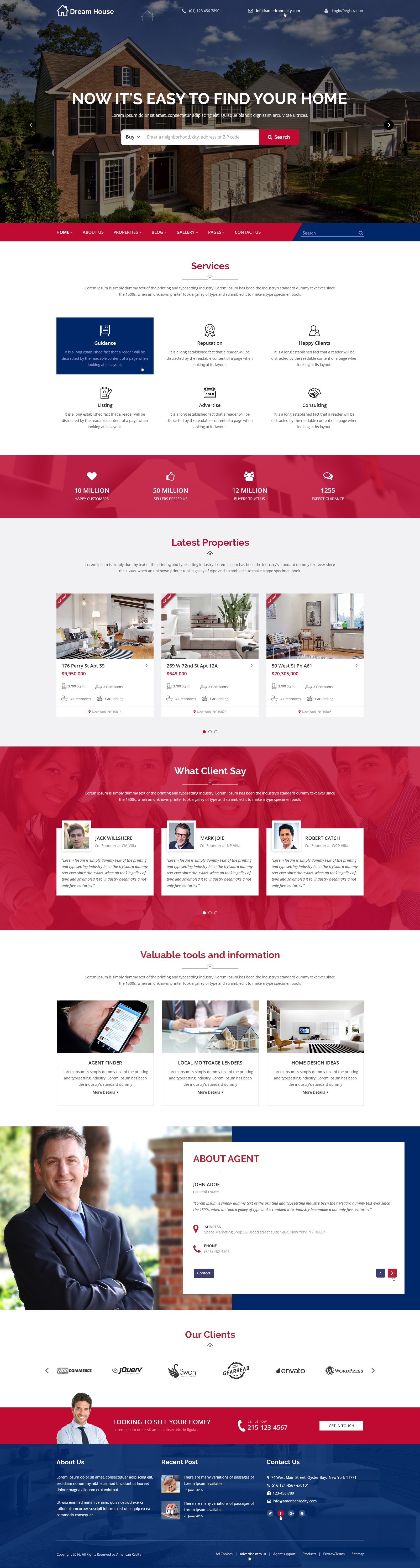A marketing image for American Reality announces "Dream House" at the top, followed by contact information: "info@AmericanReality.com" and numbers "01123456789". The photograph of a charming house below the text is complemented with the tagline, "Now it's easy to find your home." A prominent white search bar with a red search button invites users to begin their property search. 

Below this, a navigation menu offers drop-down options for "Home," "About Us," "Properties," "Blog," "Gallery," "Pages," and "Contact Us." These are displayed on a predominantly red search bar. Further down, a blue-hued section features another search bar, transitioning to a white area highlighting their services: "Guidance," "Listing," "Reputation," "Advertise," "Happy Clients," and "Consulting," each accompanied by descriptive paragraphs.

A striking red bar showcases impressive statistics: "10 million happy customers," "50 million sellers prefer us," "12 million buyers trust us," and "101,255 got expert guidance." Below this, the "Latest Properties" section displays three property listings with an option to view more through navigational dots.